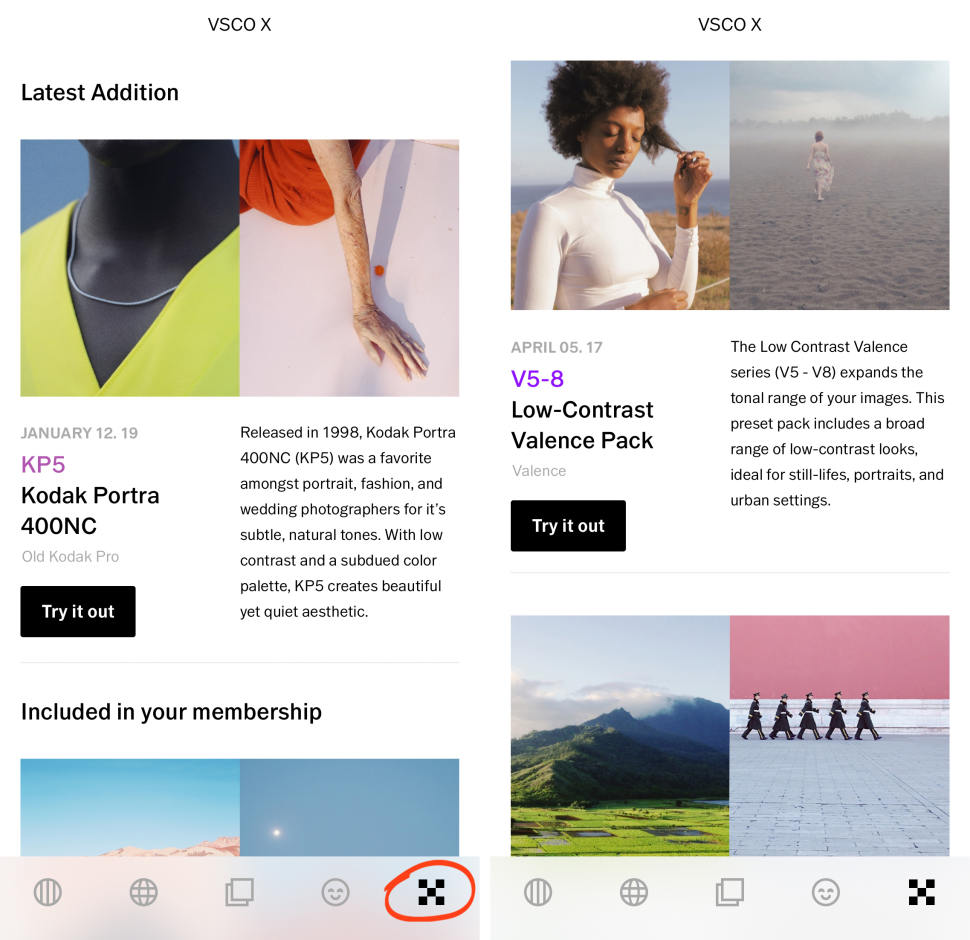The image showcases two screens displaying information about VSCO-X's latest editions of image presets.

**Screen 1:**
The first screen highlights the "VSCO-X Latest Edition." It features two sample images:
1. A mannequin dressed in a neon-colored top, accessorized with a silver necklace.
2. A person sitting upright with one hand behind their back.

Text on this screen announces the release details and features of the "Kodak Porta 400NC" preset:
- Release date: January 12, ‘19
- Description: "Released in 1998, Kodak Porta 400NC was a favorite amongst portrait, fashion, and wedding photographers for its subtle, natural tones. With low contrast and a subdued color palette, KP5 creates a beautiful yet quiet aesthetic."
- It also mentions that this preset is included in the VSCO-X membership and includes a "Try it now" button.

Additional features on this screen include a panel of five icons, with the fifth icon, which resembles five black squares, circled in red.

**Screen 2:**
The second screen also references VSCO-X, focusing on another set of presets released on April 5, '17. It details the "V5H Low Contrast Balance Pack," which is designed to expand the tonal range of images, with presets V5 through V8 offering a variety of low-contrast looks suitable for still lifes, portraits, and urban settings. This screen also includes a "Try it now" button.

Two illustrative images exemplify the effects:
1. A person wearing a white turtleneck, pulling their hair while standing outdoors under a sunny sky.
2. A black-and-white photo capturing the back of a person walking on the beach.